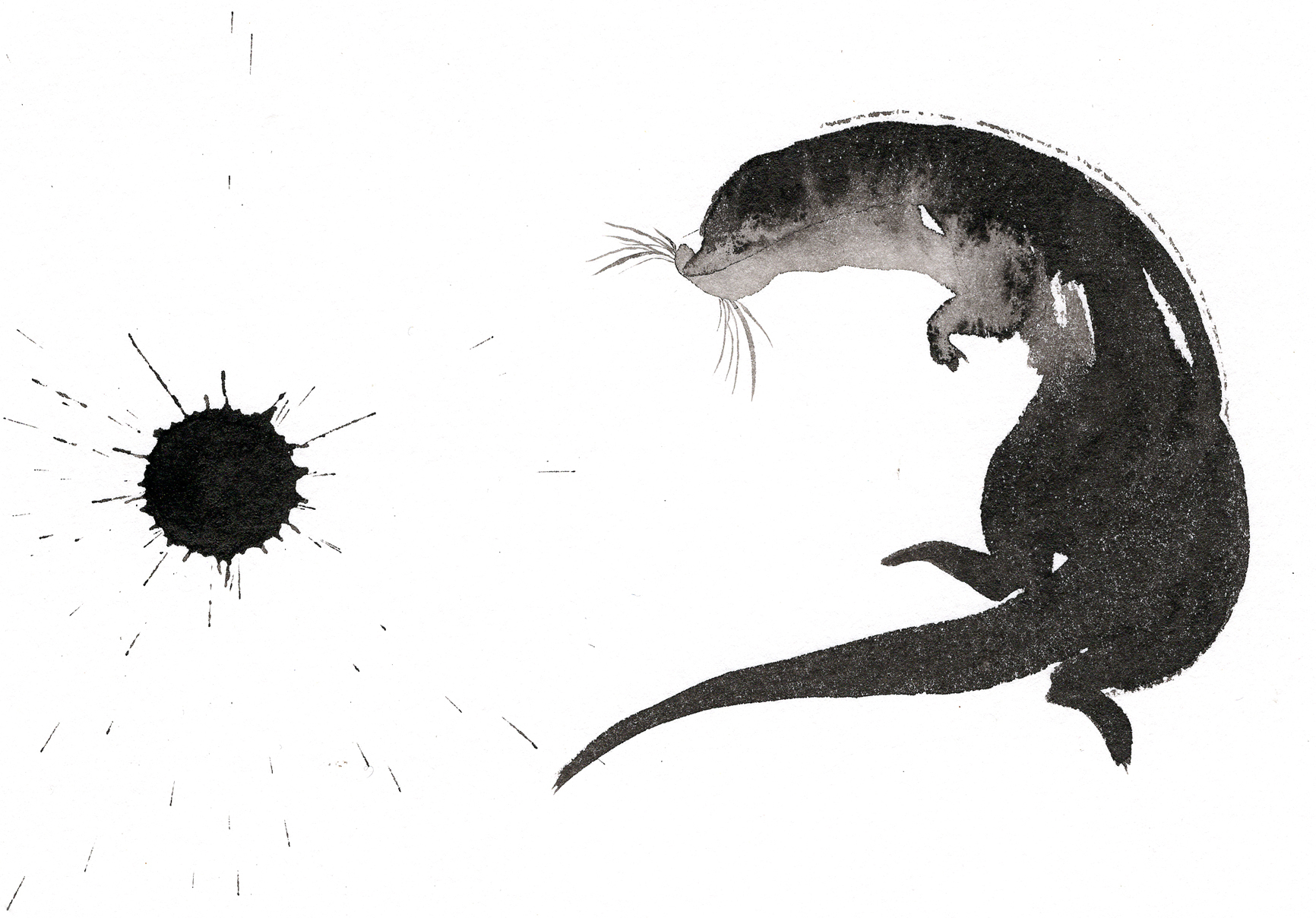The image is a rectangular watercolor painting, approximately five inches wide by four inches high, set against a completely white background. On the right side, there is a detailed illustration of an otter, depicted in shades of black, gray, and white, with a scattering of white dots on its darker areas that give it a slightly glossy appearance. The otter's body is coiled in a backward 'C' shape, with its head facing to the left, characterized by visible whiskers and a small, light gray nose. Its long tail curves back towards the left, stretching further than its head. The otter's underside is light gray, while its back is a darker gray. Visible are the left front paw situated beneath its body, and its legs and feet appear on either side of the tail below. To the left of the otter, occupying the left-hand side of the painting, is a prominent black paint splatter. This splatter is dense at its center with streaks radiating outward over the pale gray splatters in the background, creating a dynamic contrast with the detailed otter on the right.